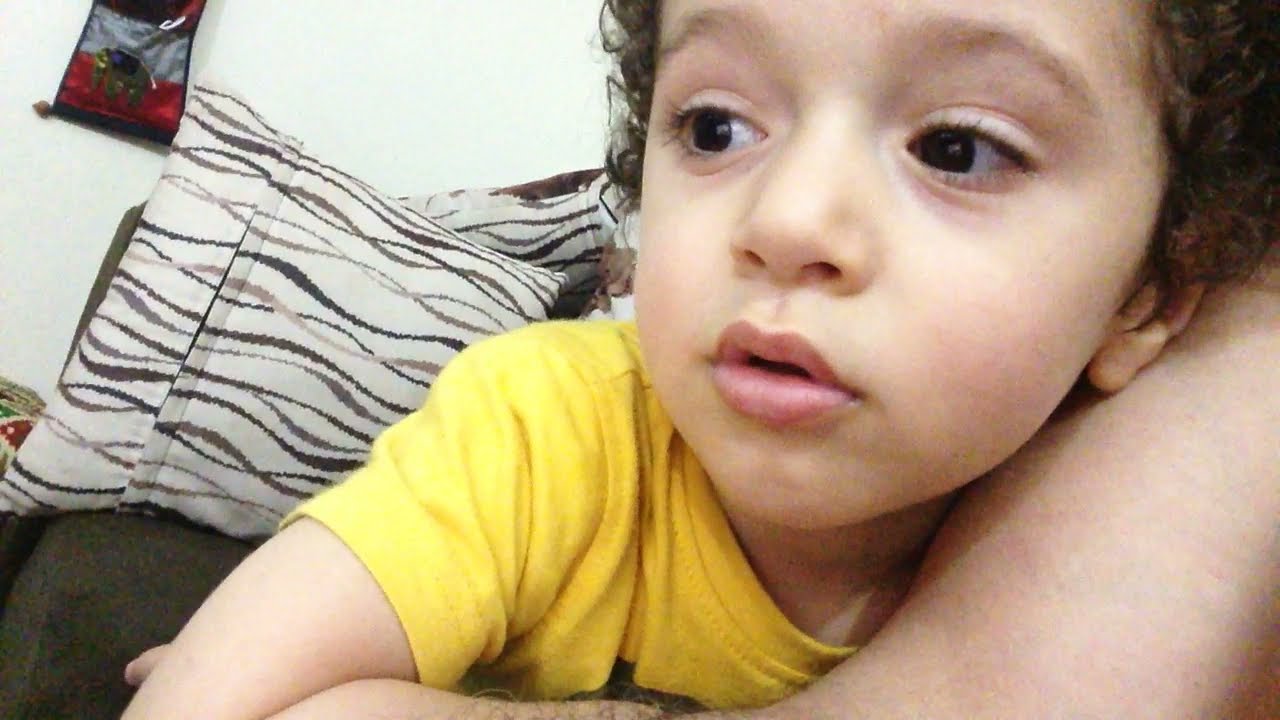The photograph features a young child, possibly a boy with olive-toned skin and brown curly hair, who looks to be either Indian or Latino. He is wearing a yellow short-sleeve t-shirt and is positioned on what appears to be a dark-colored couch. The child is lying or sitting on someone’s lap, with a light-skinned adult's smooth forearm, slightly hairy on the top, draped around him. The focal point is a close-up of the child’s face and right shoulder as he gazes to the left of the frame. Behind him, distinct white couch cushions with wavy black, tan, and brown patterns are visible, along with a white wall and a piece of artwork featuring an elephant on the far left. The serene scene is accentuated by the child's relaxed posture and the cozy, intimate setting.